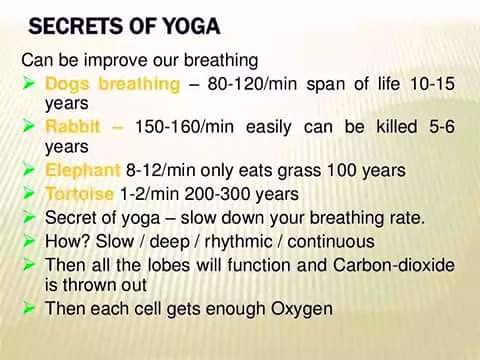The image displays an instructional graphic about the "Secrets of Yoga" in bold text at the top. Underneath, it outlines the significance of breathing rates among different animals, presented with lime green bullet points on a background of golden rays. The text highlights that dogs have a breathing rate of 80 to 120 per minute with a lifespan of 10 to 15 years, rabbits breathe 150 to 160 times per minute with a lifespan of 5 to 6 years, elephants breathe 8 to 12 times per minute and live up to 100 years on a grass diet, and tortoises breathe 1 to 2 times per minute, living up to 200 to 300 years. The graphic emphasizes that the "Secret of Yoga" is to slow down the breathing rate to achieve slow, deep, rhythmic, and continuous breaths, promoting better lung function, expelling more carbon dioxide, and ensuring each cell receives enough oxygen.